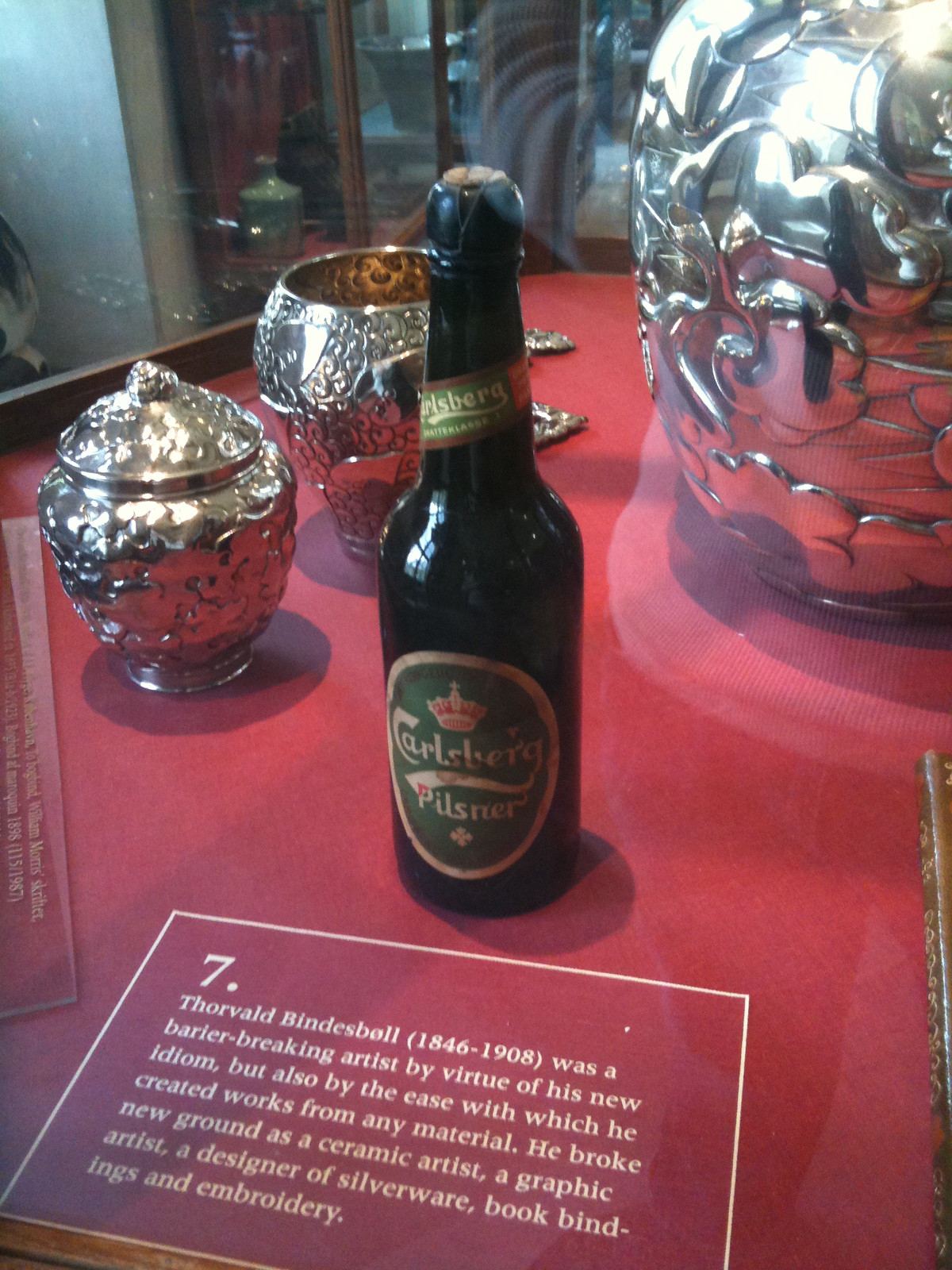The image depicts a vintage black glass bottle with a brown cork and a green label reading "Carlsberg Pilsner," situated within a glass display case. This carefully lit display features the bottle on a striking red surface. Surrounding the bottle are several sterling silver vessels, including one with a cover, another without, and a large vessel positioned in the distance. In front of the bottle, slightly angled, is a prominent red placard with a white border. The placard includes multiple lines of white text detailing the accomplishments of Thorvald Bindesbøll (1846-1908), an innovative artist celebrated for his versatility and pioneering work in ceramics, graphics, silverware design, book bindings, and embroidery.